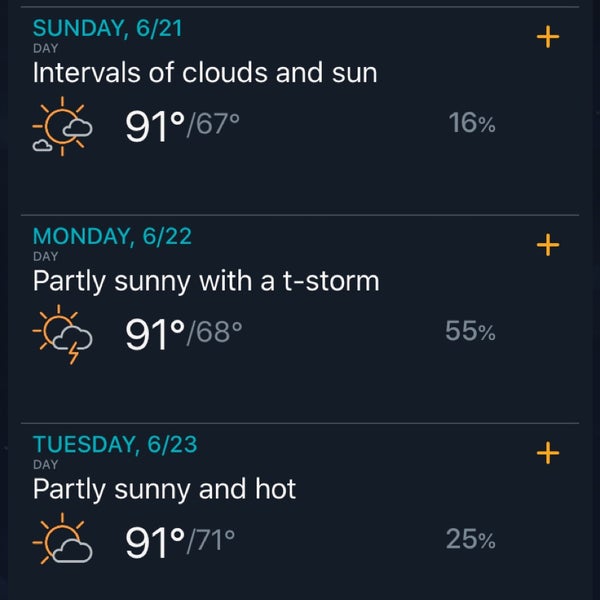A detailed caption for this image could be:

"This is a screenshot from a weather application set against a black background. At the top, blue text reads 'Sunday, 6-21, day', followed by a weather description in white letters that states 'Intervals of clouds and sun'. Accompanying this, there is an icon depicting a sun partially covered by clouds. The temperature high is noted as 91 degrees, with a low of 67 degrees, and a precipitation chance of 16%. Below this, 'Monday, 6-22, day' is displayed with a forecast of 'Partly sunny with a thunderstorm', visualized by an icon of a sun, a cloud, and a lightning bolt. The temperatures for Monday are 91 degrees high and 68 degrees low with a 55% chance of precipitation. The following day, 'Tuesday, 6-23, day', is described as 'Partly sunny and hot', represented by a sun and cloud icon. The temperature is listed as 91 degrees high and 71 degrees low with a 25% chance of precipitation. The screenshot is purely composed of text and simple weather illustrations, with no photographic elements, people, animals, birds, plants, flowers, trees, buildings, or automobiles present."